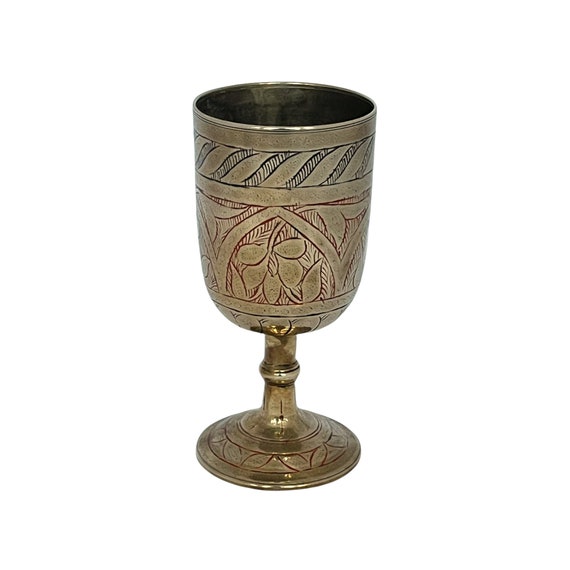This photograph features an ornate, goblet-like chalice set against a plain white background, devoid of any additional objects or shadows. The chalice itself is a reflective dark gold color with intricate designs etched into its surface. The body of the goblet showcases a detailed top pattern consisting of two horizontal lines encasing wavy blue stripes, each stripe adorned with diagonal lines crisscrossing through them. Further down, there are repeating red markings that resemble pointed archways with floral motifs inside. The base of the goblet features a red leaf-like pattern with a central notch, enhancing its elaborate design. Despite its aged appearance, it’s hard to discern if this aesthetic is stylistic or indicative of actual antiquity.